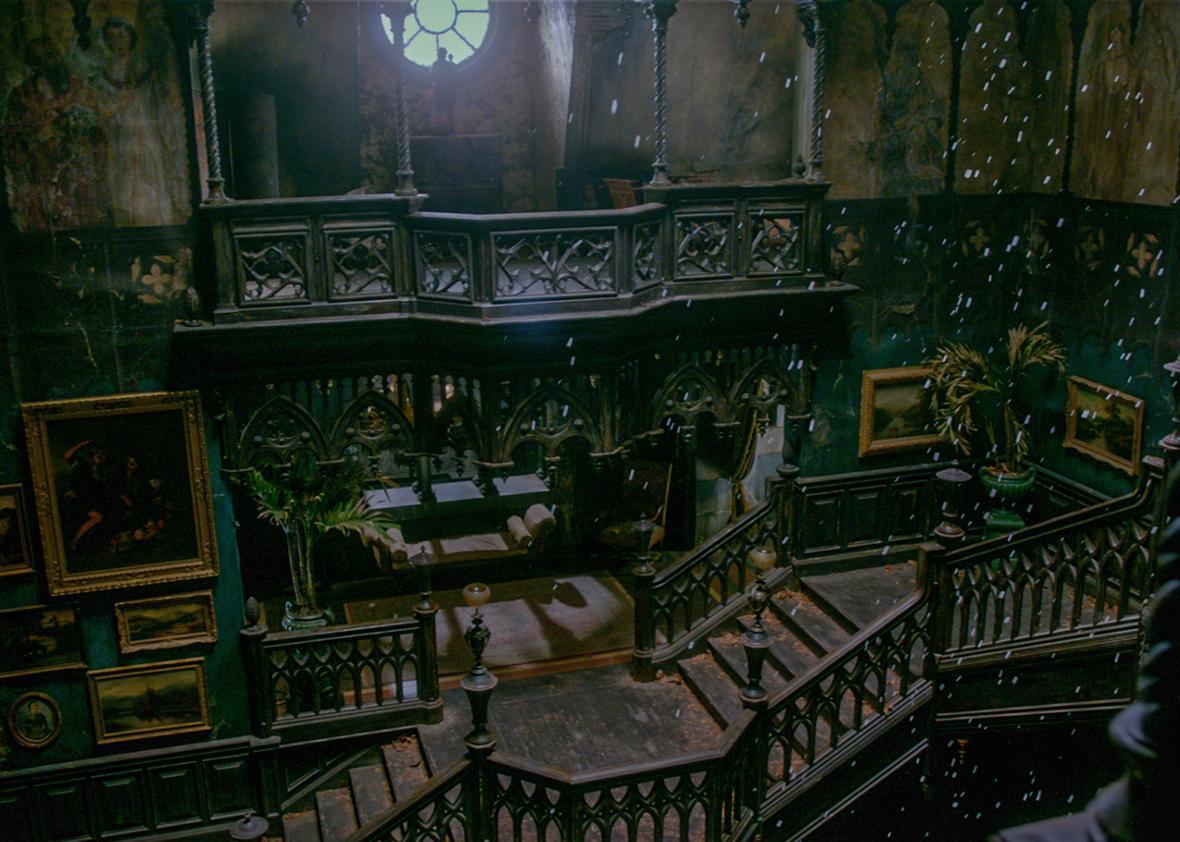The photograph showcases the dim interior of an antiquated building, evoking a sense of the Victorian era with its somber, outdated decor. The central feature is a dark brown staircase leading downstairs, flanked by an intricately carved railing adorned with leaf motifs. The walls, clad in dark panels, are dotted with gold-framed paintings and what appear to be suspended chairs, adding to the eerie ambiance reminiscent of a haunted house. Amidst this scene, specks resembling dirty air particles are visible, enhancing the gloomy atmosphere. A round window at the top of the stairwell filters in dim light, through which a shadowy figure seems to be peering out, and scattered plants add a touch of life to the otherwise dreary setting.